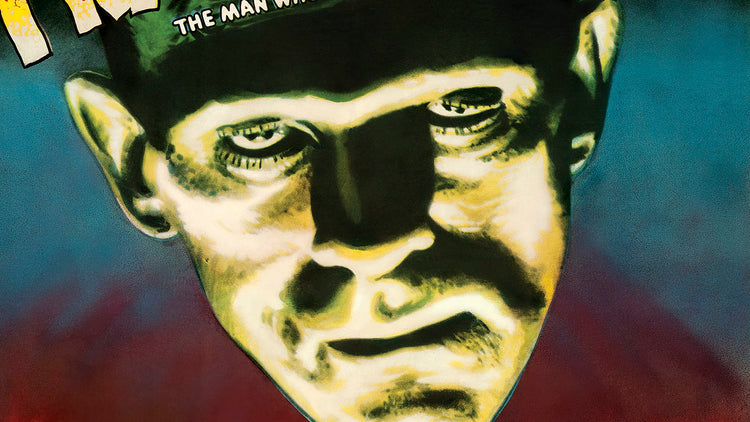This detailed photograph resembles an old movie poster, showcasing a close-up of a man's face, likely inspired by Frankenstein. The man's visage is dramatically lit from below, casting dark shadows under his eyes and across his forehead, giving it an ominous and spooky ambiance. The haunting green and white silhouette accentuates his scraggly facial hair, including a mustache and some chin hair, further enhancing the eerie effect. His heavily lidded eyes stare directly at the camera, intensifying the unsettling atmosphere.

The man’s face is predominantly green, especially in the center where his nose, forehead, and hair are immersed in a ghoulish hue, almost reminiscent of Frankenstein’s monster. The backdrop features a dark blue and purple gradient, adding to the chilling mood of the image.

Text elements in the upper left corner of the image are partially obscured, showing fragments of a larger title and a subtitle. "The Man Who" can be discerned from the subtitle, while potential letters "F," "R," and "A" hint at the larger title above. The incomplete text, coupled with the spine-chilling visual, suggests this is indeed part of a classic horror-themed poster.